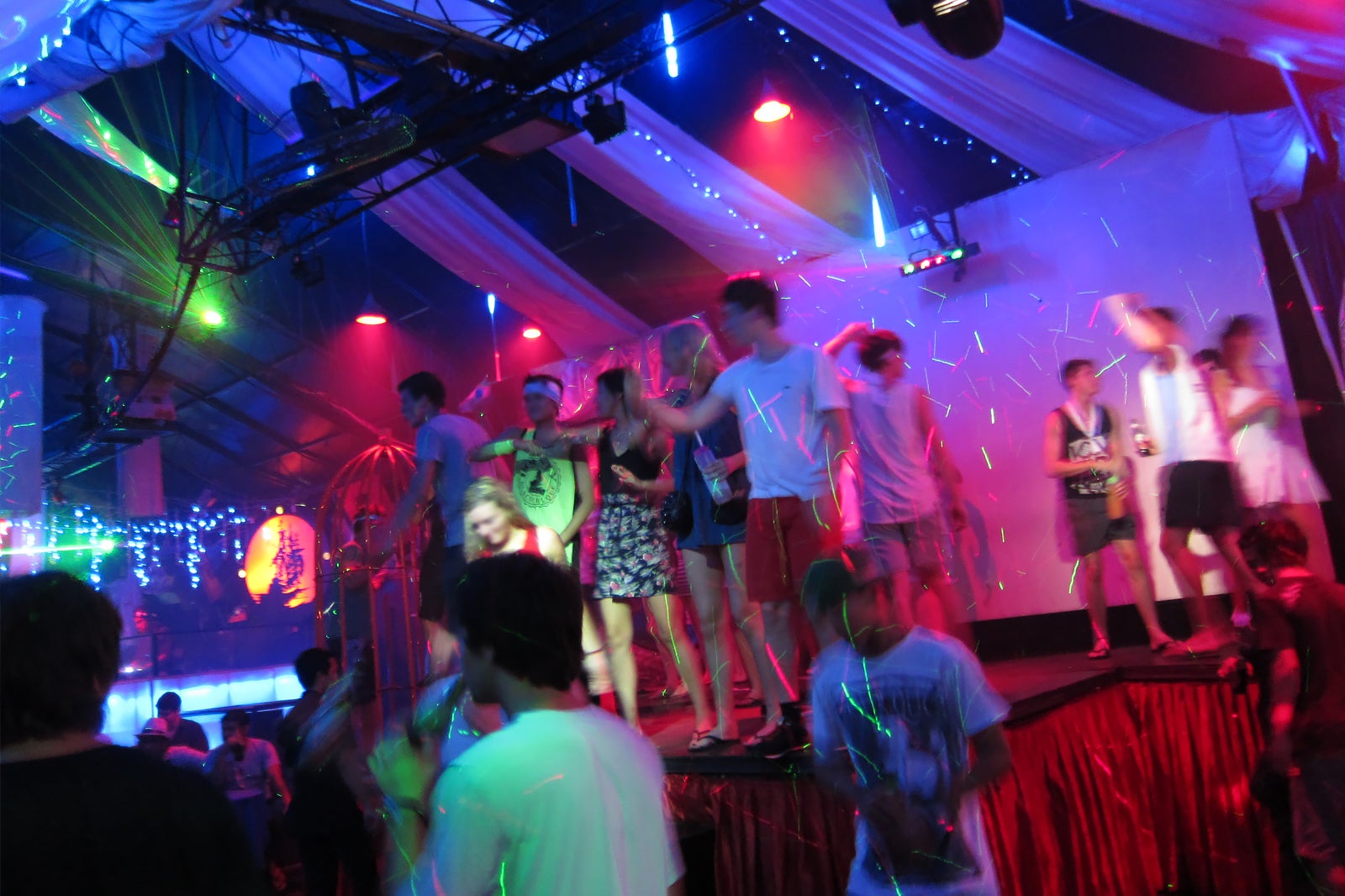The image depicts the energetic interior of a portable dance club, set up like a 70s disco haven, with an elevated stage and vibrant atmosphere. The setup features twisting, twirling laser lights and spotlights illuminating the dancers and casting dynamic patterns on the white walls. The ceiling sports racks of multicolored lights and appears tent-like, with rippling fabric and visible support structures, suggesting its temporary, portable nature.

The stage is decorated with pleated red curtains around its base, and on it stands a group of young dancers. There are about six kids to the left, dressed in various colored shirts, including a boy in a white shirt and black shorts, a child in a green shirt with a white hat, and girls in black and floral skirts. Some dancers are also on the ground, adding to the lively scene. A prominent feature is a boy in a white shirt with a black design, positioned centrally and facing the camera.

Red and green lights beam down on the dancers, who are surrounded by the purple walls of the stage and silhouetted against reflections from a waterway outside the building. The reflections capture the glimmering city lights, complementing the flashes of light from what appears to be sparklers held by some of the attendees. The entire scene exudes the festive and electric vibe of a mobile discotheque, brimming with youthful energy.